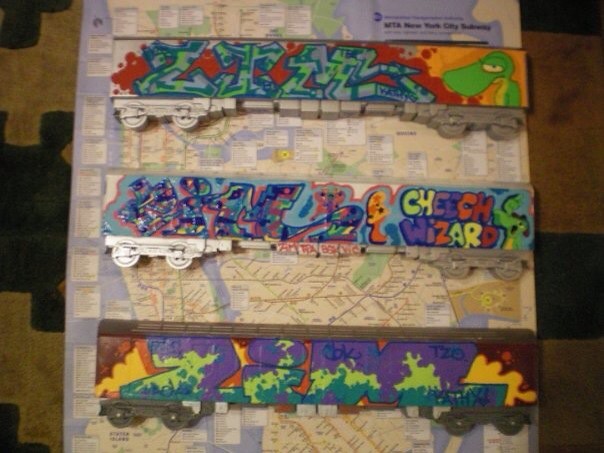The image features three intricately detailed model trains, each creatively adorned with colorful graffiti, set atop a New York City subway map. The train cars, which have wheels and trucks at both ends, bear vivid graffiti in hues of purple, green, blue, red, and orange. Among the graffiti are images of an alien or lizard-like creature and various words, including "Cheech Wizard" prominently displayed in multicolored lettering and "ZTM" and "DSM" in purple and green. The subway map beneath the models is detailed with the city's essential MTA transit lines in yellow, white, blue, green, red, and black, identifiable by their unique colors and labels. This artistic arrangement appears to be carefully laid out on a flat surface, resembling a table or floor.